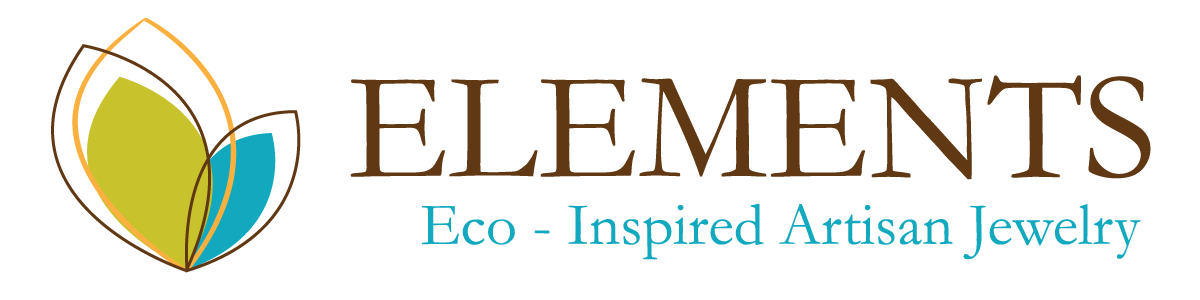The image displays a sign set against a white background featuring an artistic logo and descriptive text. On the left side, there are three outlined leaf-shaped graphics. Two of these leaves are partially filled with color: one leaf is filled with green and tapers towards the top left, while the other is blue and inclines to the top right. The green leaf has a light red border, and the blue leaf has an orange border. Additionally, a third leaf outlined in white is present. To the right of these graphics, in large dark brown capitals, is the word "ELEMENTS." Below this, smaller, centered text in baby blue reads "Eco-Inspired Artisan Jewelry," with only the first letters of each word capitalized. The overall design communicates a clean, eco-friendly aesthetic for a business specializing in artisan jewelry.